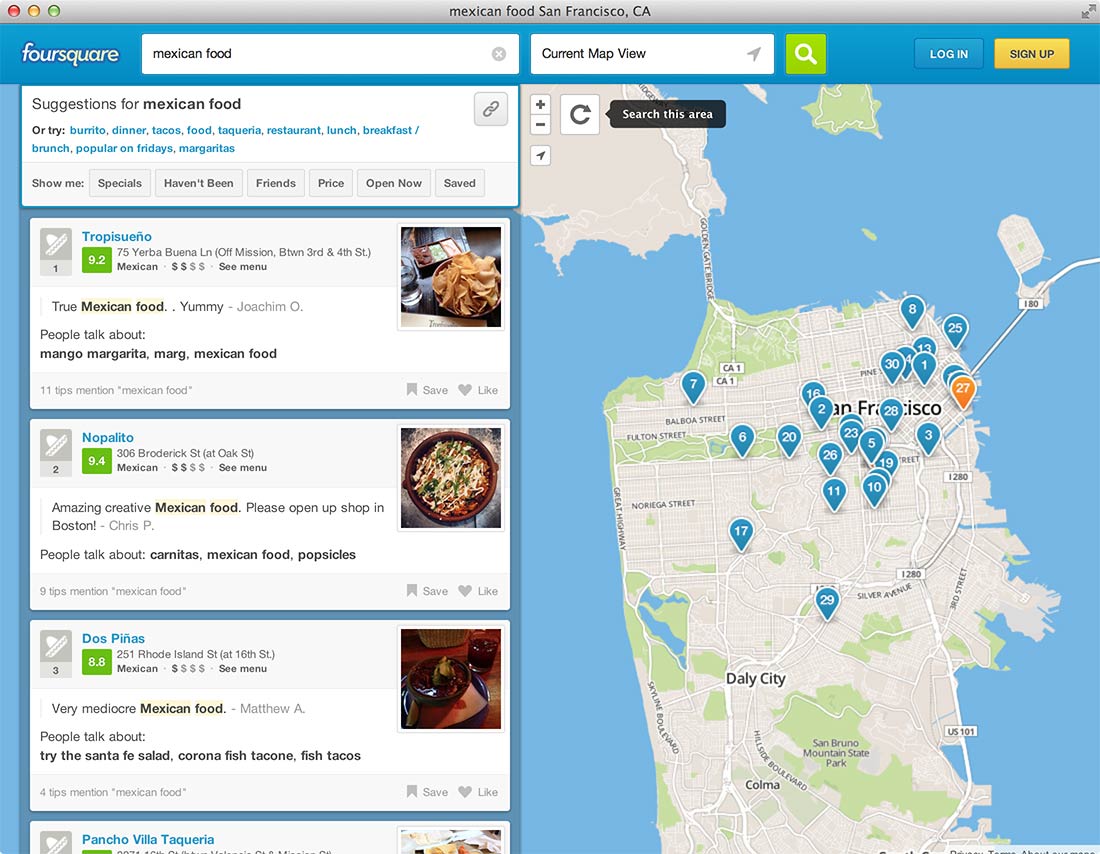This image captures a web page designed for finding Mexican food in San Francisco, California. At the top, a gray navigation bar features red, yellow, and green circular icons on the left, resembling browser window controls. Centrally within this gray bar, the text "Mexican food, San Francisco, California" is displayed. On the right side, there are two arrows pointing up and down.

Just below, a blue bar branded with "Foursquare" accompanies a search bar pre-filled with "Mexican food." Adjacent to this, the text "Current Map View" is displayed alongside a green square icon with a magnifying glass. On the far right, there are two buttons for user actions: a blue "Login" button and a yellow "Sign Up" button.

The left-hand sidebar lists suggestions for specific Mexican dishes and experiences under options like "Burrito," "Dinner," and "Tacos." Directly below, a listing of Mexican restaurants is presented. The visible listings include "Trapasueño" (True Mexican Food), "No Palito" (Amazing Creative Mexican Food), "Dos Piñas" (Very Mediocre Mexican Food), and "Pancho Villa Taqueria," though full reviews are not readable in this view. It is implied that more listings are available beyond the visible three.

On the right side of the page, a map of San Francisco prominently displays markers for approximately 29 different Mexican food restaurants, assisting users in visualizing their options across the city.